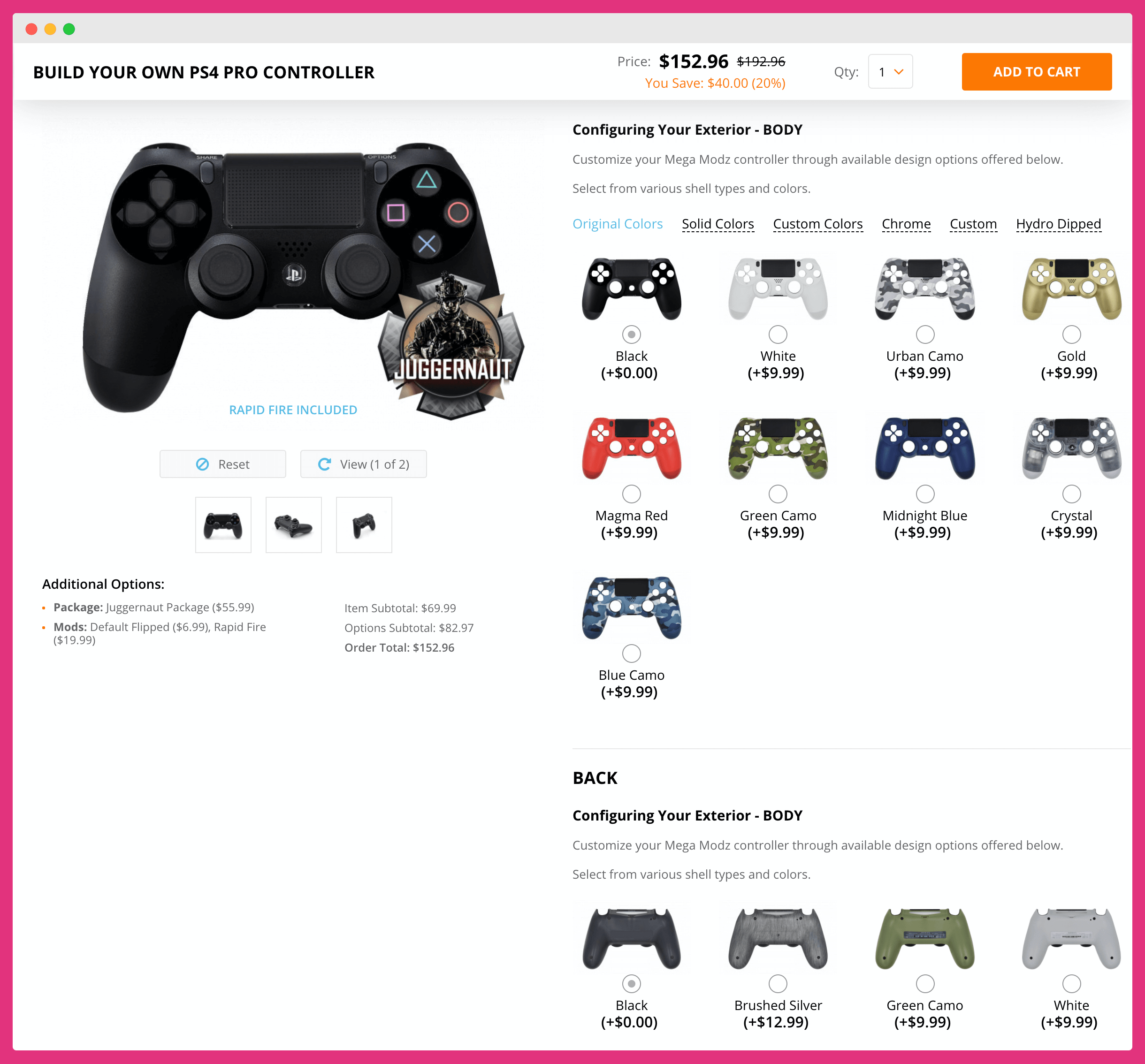This screenshot displays a web page for customizing a PlayStation 4 Pro controller. At the top of the page, there's a header that reads, "Build Your Own PS4 Pro Controller." On the left side, the current price of $152.96 is prominently displayed, reduced from the original price of $192.96. A note in red indicates that customers save $40 or 20%. Below this, there is a quantity selector set to one, followed by an "Add to Cart" button.

To the left, there’s an image of a black PS4 controller labeled "Juggernaut" above an icon. Adjacent to this are a reset button and a "View 1 of 2" button, with three small thumbnails showcasing different angles of the black controller. Beneath these thumbnails, there are additional customization options, though some text is illegible.

On the right side, the section titled "Configuring Your Exterior Body" describes the process of customizing the "Mega Mode" controller through various design options. There are nine shell types and colors available: Black, White, Urban Camo, Gold, Magma Red, Green Camo, Midnight Blue, Crystal, and Blue Camo. Additionally, the back of the controller can be customized with choices like Black, Brush Silver, Green Camo, and White.

This detailed layout provides a comprehensive overview of the customizable features available for the PS4 Pro controller.